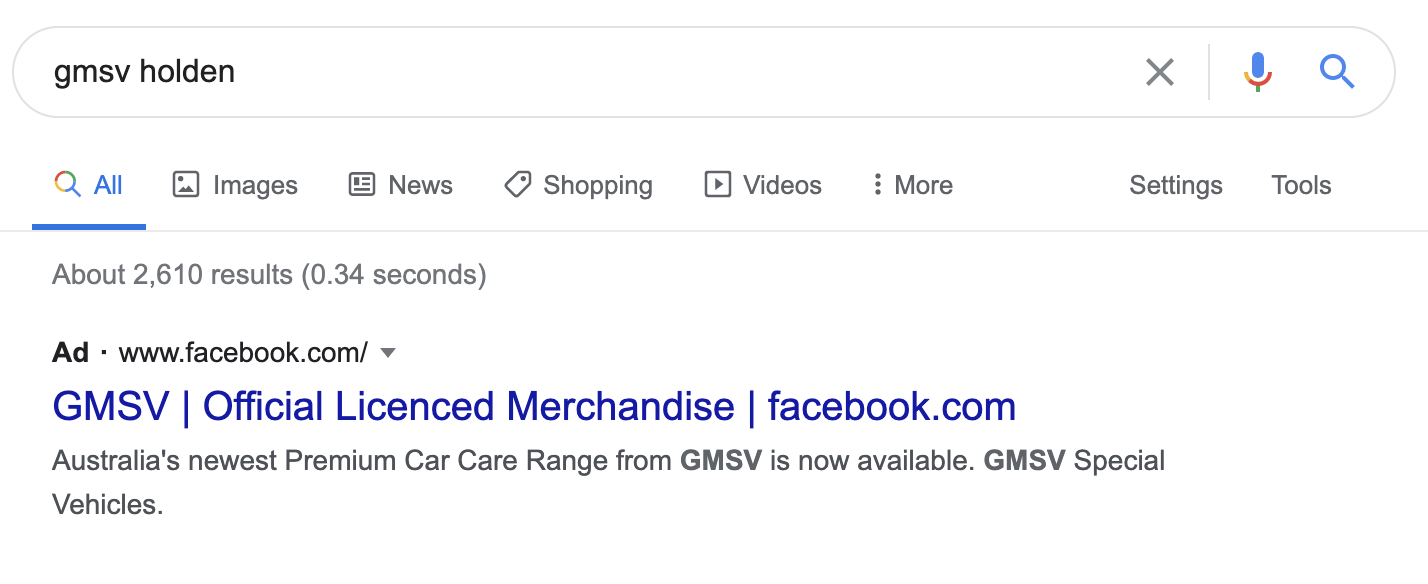The image displays a Google search results page with a clean, white background. At the top, there is a text box labeled "search box" where the phrase "GMSV Holden" is entered. To the right of this box, there are three icons: an "X," a microphone, and a magnifying glass.

Below the search box, there is a navigation bar with the options "All," "Images," "News," "Shopping," "Videos," "More," "Settings," and "Tools." A light gray line runs horizontally across the page beneath these options, with a dark blue segment directly under the "All" tab, indicating that the "All" section is currently selected.

The next section displays the search results statistics, noting that there are approximately 2,610 results found in 0.34 seconds.

The first search result is a link to Facebook, with the URL "www.facebook.com" listed. It appears as "GMSV Official Licensed Merchandise" and is connected to GMSV's official Facebook page. The text below this link describes Australia's newest premier car carrier range from GMSV as now available.